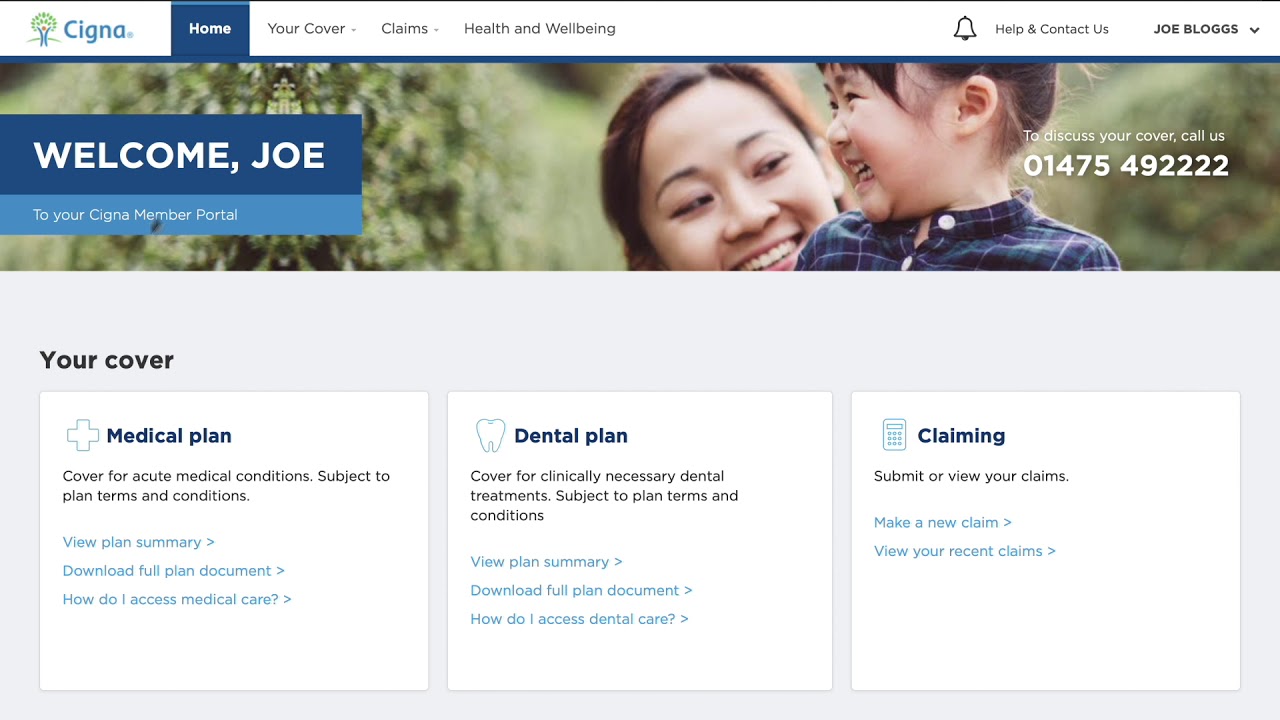A detailed screenshot of someone's Cigna member portal is displayed. At the top, there is a white border with the Cigna logo on the left, featuring the word 'Cigna' in blue and a tree icon beside it. The navigation menu includes sections such as Home, Your Cover, Claims, and Health and Well-being, with 'Home' currently selected.

Directly below, there is a narrow banner image portraying an Asian woman and her child. To the left of this image, a rectangular box with a gradient background from dark blue to light blue welcomes the user: "Welcome, Joe, to your Cigna Member Portal" in white text.

Below this, the main content area has a gray background featuring three white-bordered squares, each representing different sections of coverage. The area is titled 'Your Cover'. 

- The first square is labeled 'Medical Plan', detailing coverage for acute medical conditions subject to plan terms and conditions. It provides three options: 'View Plan Summary', 'Download Full Plan Document', and 'How Do I Access Medical Care'.

- The second square is titled 'Dental Plan', covering clinically necessary dental treatment, also subject to plan terms and conditions, with similar options: 'Summary', 'Download', and 'How Do I Access'.

- The third square is labeled 'Claiming' and allows users to submit or view their claims, offering choices to 'Make a New Claim' or 'View Your Recent Claims'.